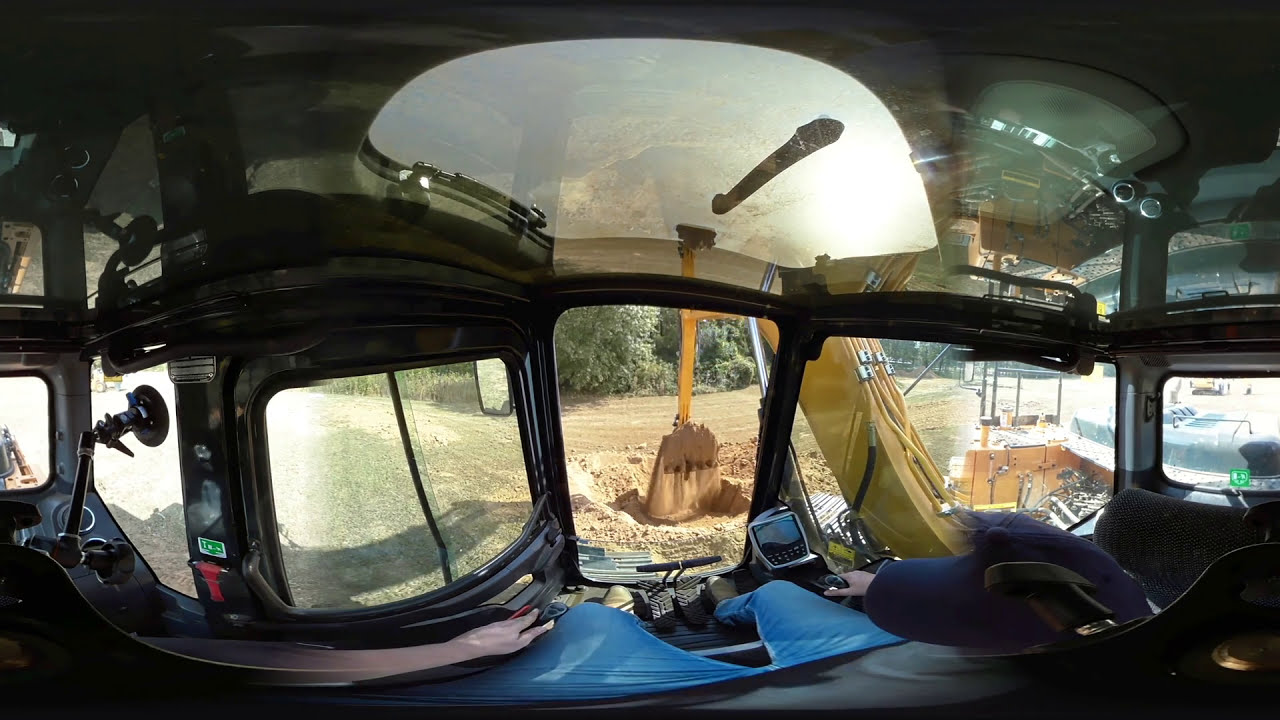The image depicts the interior of a large, yellow construction excavator in active use. Positioned centrally and slightly towards the right is the operator, dressed in a dark blue shirt or jacket and light blue jeans. His right hand manipulates the machinery's control lever situated near a small monitor or view screen, while his left hand rests casually to the side. The operator's foot is engaged with a pedal on the vehicle's floor. The cabin's design features several windows, including a main windshield and a larger overhead window, allowing for clear visibility. Outside, the excavator’s prominent hydraulic arm, topped with a scooper bucket, digs into a patch of dry, brown earth, possibly sand, surrounded by a few trees in the background. On the far right of the image, the edge of a window with a brownish-black stick and a red latch is visible. The scene vividly captures the intense focus and functionality within the excavator’s cabin as it moves earth efficiently.